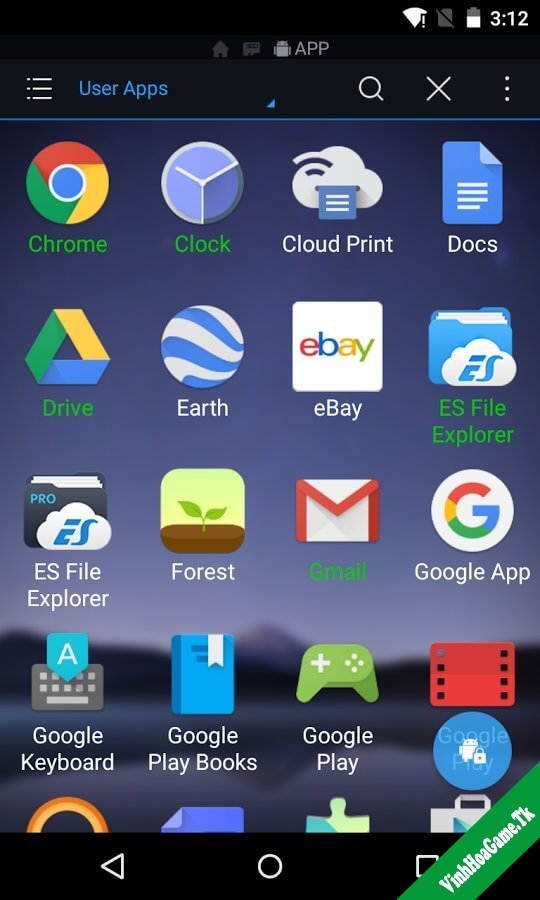In this vertically-oriented rectangular image, the screen of a device, possibly an iPad or an iPhone, is displayed with a blue background. At the top left of the screen, the text "User Apps" is prominently shown in blue print. Below this heading, there are several rows of app icons arranged from left to right. 

The first row features icons for the following apps: Chrome, Clock, Cloud Print, and Docs. The second row below includes icons for Google Drive, Earth, eBay, and ES File Explorer. The third row again shows ES File Explorer, followed by Forest, Gmail, and the Google App. In the next row, there are icons for Google Keyboard, Google Play Books, Google Play, and an additional Google Play icon which has a small lock and a robot symbol.

Towards the bottom of the screen, partial views of several icons are visible: the top portion of an orange semi-circle, the edge of a blue page, a yellow and green puzzle piece, and the top part of a shopping bag icon. In the lower right corner, running horizontally in white print, the text "vinhoagame.tk" can be seen.